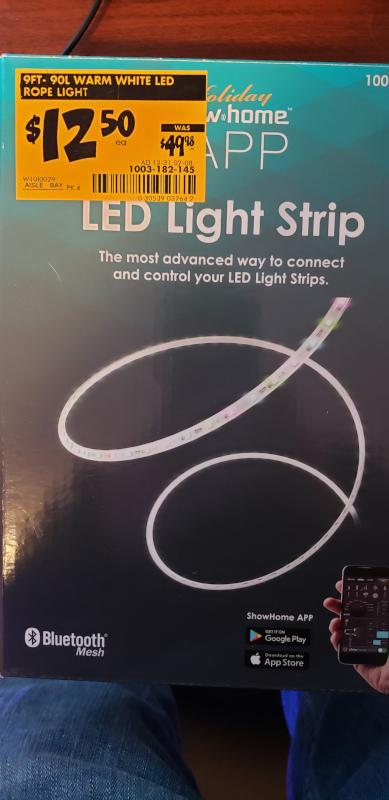This image features a boxed item for sale at Home Depot: a Warm White LED Rope Light. The box prominently displays a sale price of $12.50, marked down from $49.98. The product description on the box highlights it as the "most advanced way to connect and control your LED light strips." The featured LED light strip is depicted looping in a smooth, serpentine fashion against an eye-catching ombre background transitioning from teal to black.

In the lower left corner, the box advertises Bluetooth Mesh technology, indicating that the light strip can be connected via Bluetooth. On the bottom right, there is an image of a hand holding a smartphone alongside icons for the Home App, which is available on both Google Play and the App Store, suggesting that users can control the light strip through an app on their phone. Additionally, the upper right corner features the number "100" in white text, though its significance is unclear.

The box is resting on someone's lap, and the presence of denim-clad legs suggests they are wearing jeans.

This thorough and detailed packaging description underscores both the technological features and the aesthetic presentation of the LED rope light.